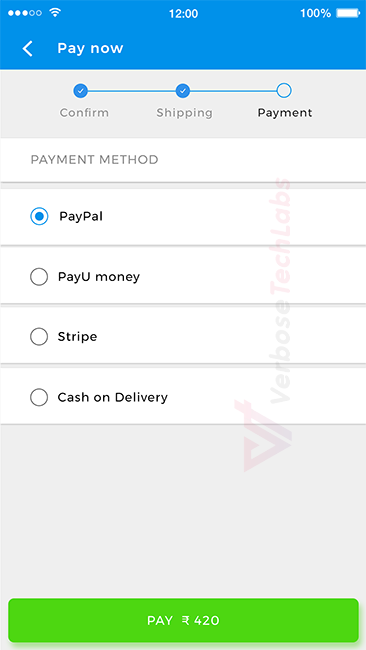A screenshot from a tablet displaying the payment stage of a purchase transaction. The interface features a predominantly white background with a medium blue banner at the top. The banner includes a white "Pay Now" heading and a left-facing arrow, allowing users to navigate back to the previous screen.

Beneath the banner, a horizontal progress indicator shows the steps of the transaction. The "Confirm" and "Shipping" steps are checked off, indicating their completion, while the "Payment" step is currently active. 

The available payment methods are listed in a left-aligned, vertical layout: PayPal, PayU Money, Stripe, and Cash on Delivery. Each option has a corresponding selection button to its left, with PayPal currently selected.

At the bottom of the screen, there is a wide, lime green "Pay" button spanning the width of the screen. The button's white text appears stretched horizontally and reads "Pay 420." The currency symbol is indistinguishable, somewhat resembling a backward euro symbol, making it unclear which currency is being used. The text's distortion adds to the ambiguity.

Overall, this image captures a critical stage in a digital transaction process, highlighting the active selection of payment method and awaiting final confirmation to complete the payment.